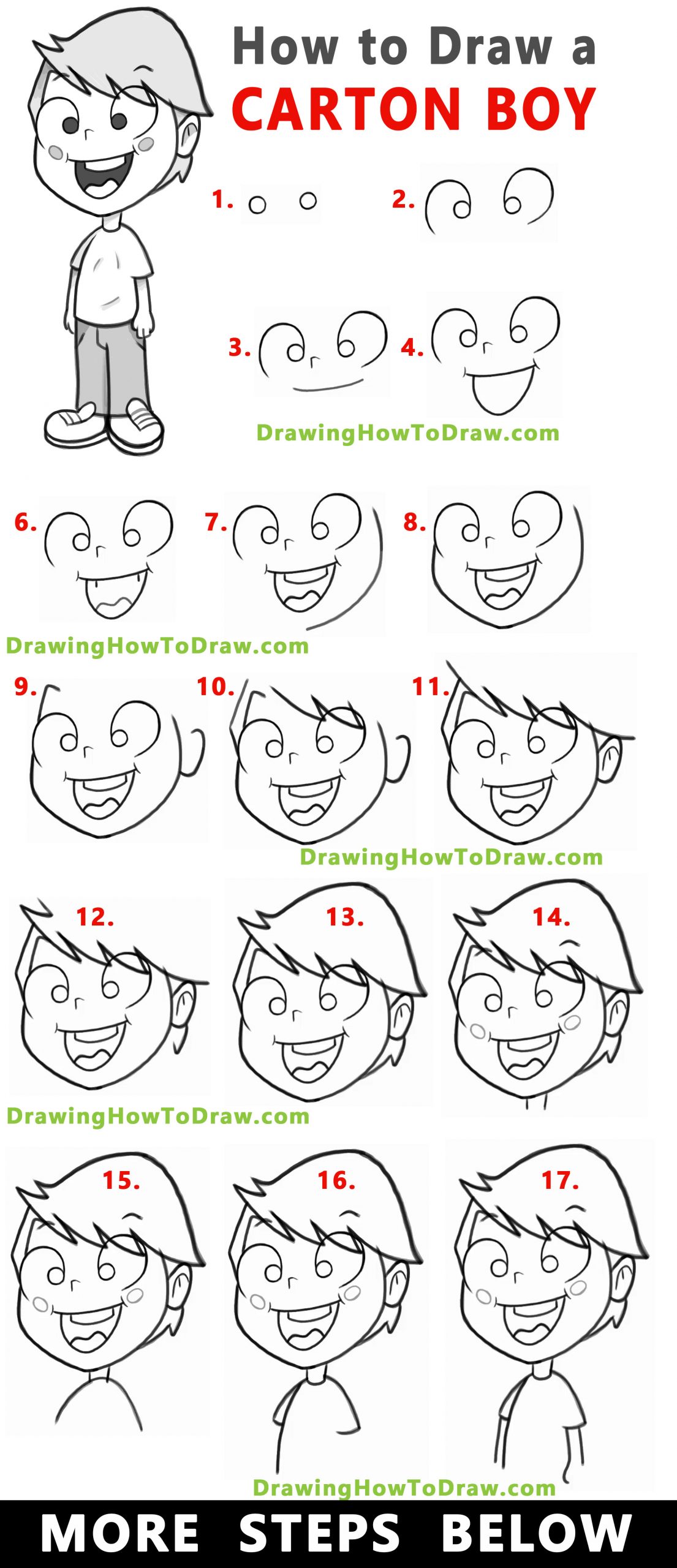This image serves as a step-by-step guide titled "How to Draw a Cartoon Boy," complete with 17 detailed steps. At the top left, there is an illustration of the finished cartoon boy, showcasing the final product. The instructions start simply with basic shapes like circles and lines to form the eyes and face, progressively adding more details like hair, facial features, a neck, and eventually the body, shirt, arms, and hands. Each step builds on the previous one, making it accessible for beginners. The guide is watermarked at intervals with "drawinghowtodraw.com," indicating the source of the tutorial. At the bottom of the image, a black bar with white text states "More Steps Below," suggesting additional instructions may follow. The entire guide is set against a white background and aims to make the drawing process easy to follow.